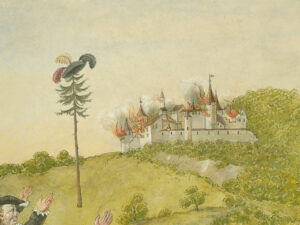A small, somewhat squarish image, likely a painting or drawing, showcases a scene dominated by a white castle with beige rooftops and multiple towers, perched on a mountain amid vibrant greenery of grass and trees. The backdrop is a cloudy, almost white sky. In the foreground, particularly in the lower-left corner, a man in a black outfit with white cuffs stands with his arms raised, looking towards the castle. Nearby, a tree, possibly a pine, has a black hat adorned with feathers—one black feather jutting to the right, a red feather to the left, and a yellow feather on top—perched atop it. This suggests the hat was blown there, and the man along with at least one other person, whose raised hands are partially visible, appears to be contemplating how to retrieve it. The castle itself seems engulfed in orange flames and thick smoke, adding a dramatic sense of urgency to the scene.